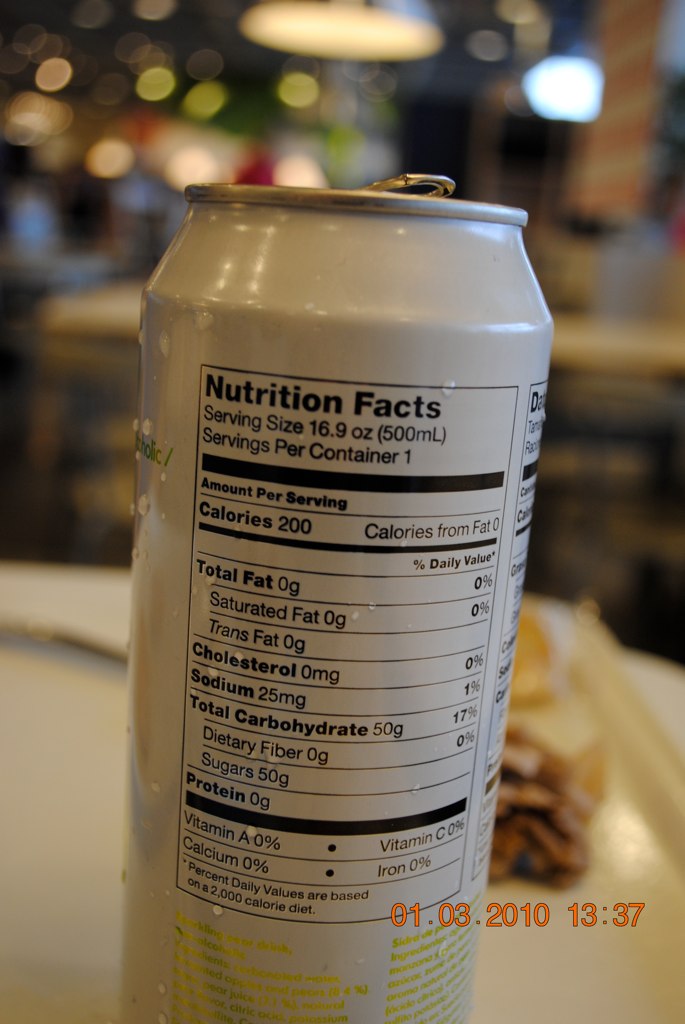This image features a tall, slender can that diverges from the typical soda can dimensions, reminiscent of those used for certain energy drinks. The can's silver top is equipped with an opened tab that slightly juts over the edge of the top rim, which is clearly visible due to the camera's low-angle perspective. The focal point of the image is the nutritional information printed in black on the white surface of the can. Additional yellow text is visible at the bottom, providing more detailed information. A date and time stamp, "01.03.2010, 13:37," is also discernible on the can.

The background features a white table surface with what appears to be some food items—possibly white bread with a darker food item or a sandwich of some kind—situated behind the can. The backdrop suggests an outdoor setting, likely an open-air restaurant, as indicated by blurred elements such as string lighting with white and yellow bulbs and a mysterious blue light. The overall scene evokes a bustling, street-like atmosphere that is lively yet indistinct due to the blurred surroundings.